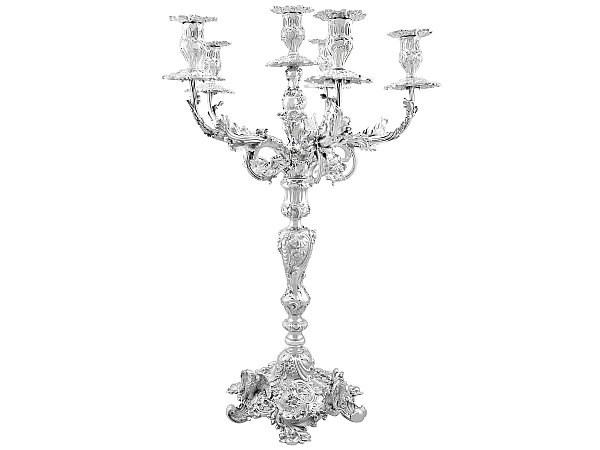This photorealistic image displays a tall, ornate candelabra set against a plain white background. The silver-colored candelabra stands centered, with a wide, intricately decorated base that narrows into a slender, heavily embellished stem. The decorative elements, which seem to include floral and vine-like patterns as well as leaves, give the piece a Victorian aesthetic. The candelabra branches into six arms near the top, though some are partially obscured. Each arm features a raised platform designed to hold a tapered candle, though the candles are absent in this image. The base is square and deeply engraved, enhancing the detailed, filigree-like ornamentation that covers the entire piece.